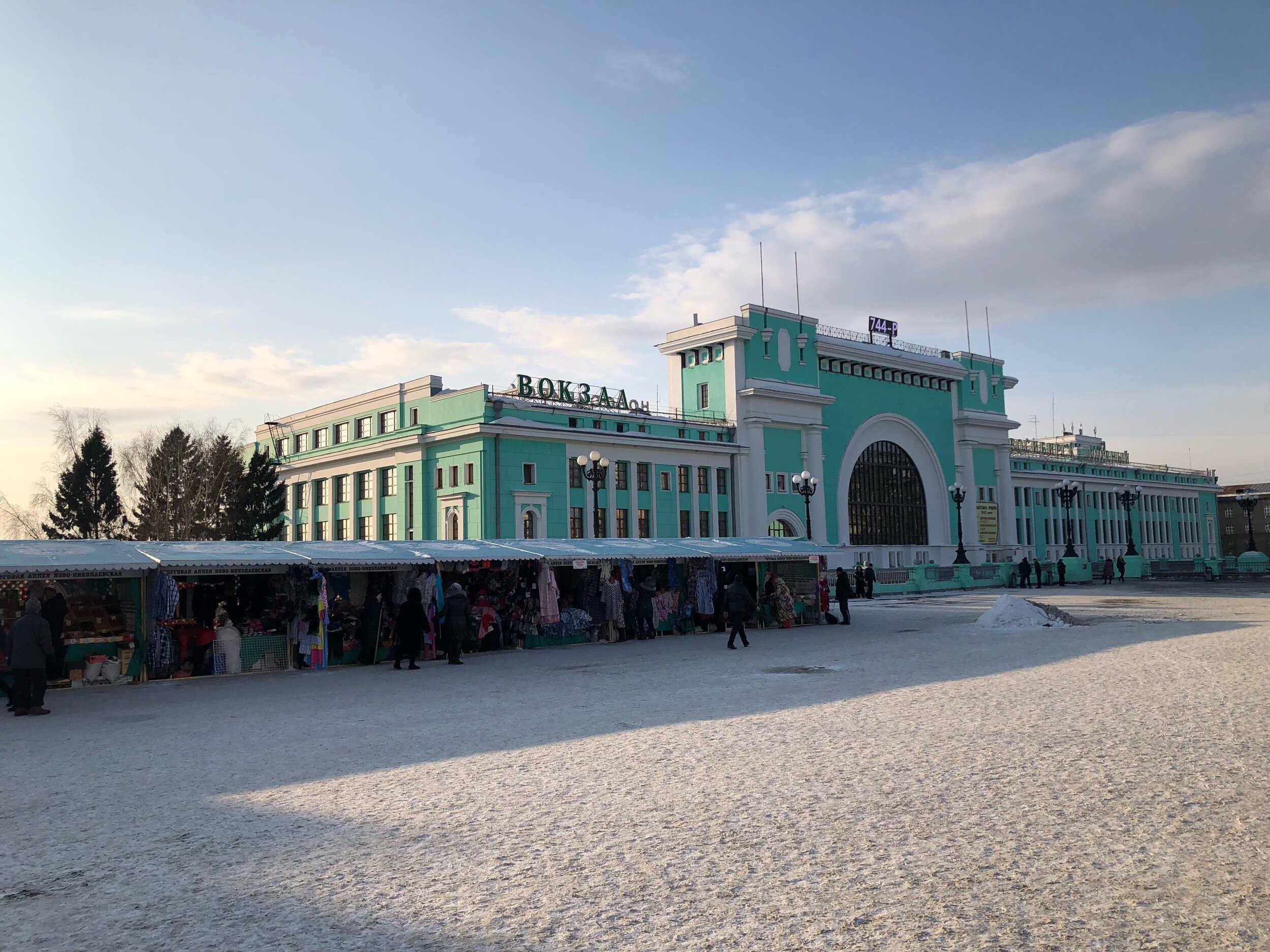In this vibrant daytime image, a bustling town center comes to life under a bright blue sky with clouds gathering on the far right. At the heart of the scene stands a large, teal-hued building reminiscent of a castle, adorned with multiple stories of windows. The building features prominent text at the top that appears to be in a Russian script, with the characters B-O-K-3-A-A visible. Surrounding the building is an active market area, featuring numerous metal-roofed vendor stalls aligned along the rough, asphalt textured ground. Crowds of people weave between the stalls, browsing through items like clothing hung up on display. The overall atmosphere is lively with a mix of people walking around, framed by lampposts in front of this grand edifice.